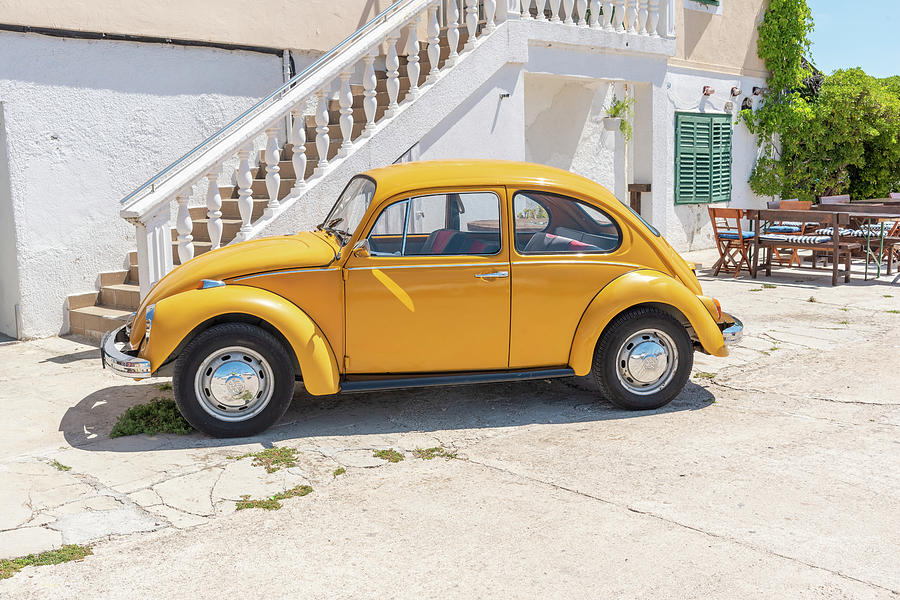This image captures an old-time, vintage yellow buggy, closely resembling a classic Volkswagen Beetle from the late 60s to early 70s, parked outside a large, concrete villa-like residence. The car, with its distinctive yellow hue and red and black seats, features black circular tires with silver hubcaps and accents along the bumpers. Notably, the car has front doors only, requiring backseat passengers to climb in. The setting suggests a European countryside location, possibly a working farm or winery, with neutral tones in the backdrop that contrast with the car’s brightness. The house, characterized by a long white railing, concrete stairs, and a sunlit atmosphere, has green windows on the right side, where wooden seats with cushions are placed. Vines grow along the house, and bits of grass and shrubbery peek through cracks in the concrete beneath the car.